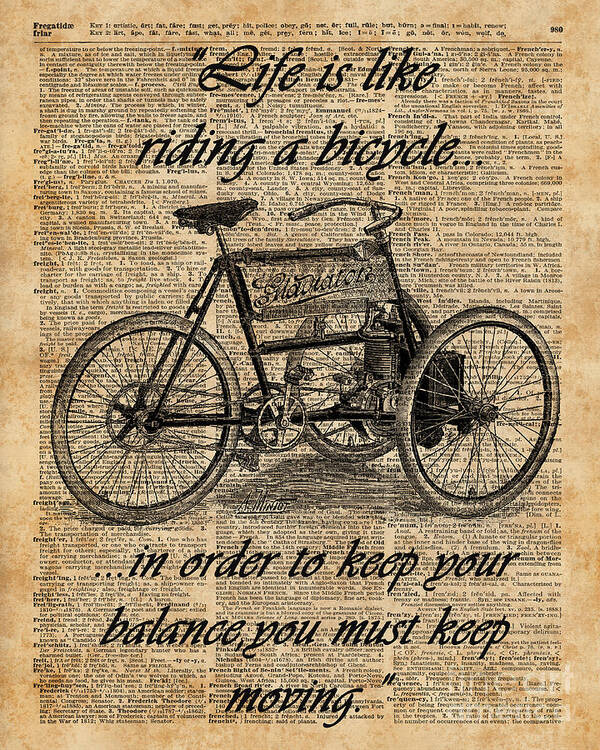The image depicts a page that resembles an old newspaper or magazine, characterized by a white and brownish hue with yellow staining indicative of aging. The background of the page is filled with three columns of illegible text. Dominating the center of the page is a detailed black-and-white illustration of a vintage three-wheeled bicycle, labeled indistinctly, but possibly starting with the letter 'G' and likely named "Gladiator."

Above and below the bicycle, a motivational quote is split into two parts, elegantly inscribed in black, fancy font:

"Life is like riding a bicycle...  
[in the middle, the image of the bicycle]  
...in order to keep your balance, you must keep moving."

The tricycle's old-fashioned style, potentially from the early 1900s, adds a nostalgic touch to the composition, though its connection to the message remains somewhat ambiguous.